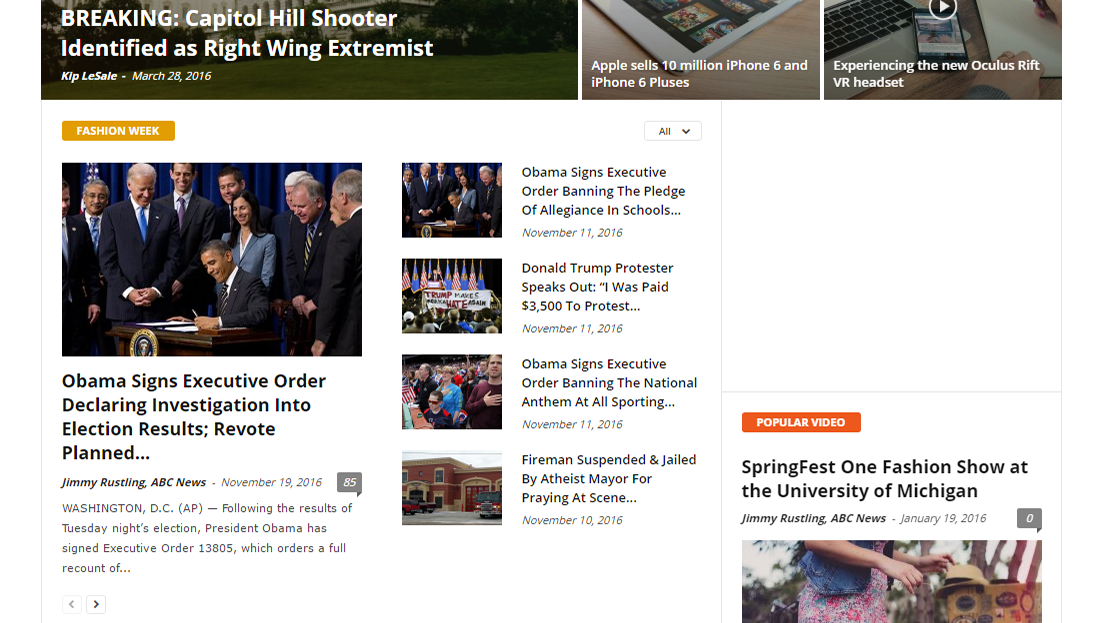The following image captures a busy web page filled with various articles and multimedia elements. 

### Central Image
At the center of the page is a significant photograph depicting Barack Obama standing alongside Joe Biden, presumably taken during Obama's presidency, surrounded by numerous congressmen. The focal headline directly beneath the image reads, "Obama signs executive order declaring investigation into electoral results, re-vote planned..." The text below attributes the news to Jimmy Wrestling of ABC News, dated November 19, 2016, from Washington, D.C. (AP). It further explains that following the outcomes of the Tuesday night election, President Obama has signed Executive Order 13805, mandating a complete recount of the votes, though this text trails off with ellipses.

### Navigation and Header
Above the central image, in bold white text, the header states "Breaking... Capitol Hill shooter identified as right-wing extremist." The page features navigation arrows, with the left arrow grayed out indicating an inability to go back, and the right arrow molded to suggest forward navigation, both housed within a square.

### Sidebar Content
- **Left Sidebar:** Features a prominent name, "KIP Leslie LeSale," with the date March 28, 2016.
- **Right Sidebar:** Displays an array of devices and articles. The top part has an image of a white Apple tablet with the text "Apple sells 10 million iPhone 6 and iPhone 6 Pluses." Adjacent to it is a smartphone screen showcasing an app that advertises the new Oculus Rift VR headset.

### Additional Articles
The right sidebar continues with further images and headlines:
1. **Obama with Congress (Repeated):** Similar to the central article, but with the headline reading "Obama signs executive order banning the pledge of allegiance in schools..." dated November 11, 2016.
2. **Protestors with American Flags:** Captioned "Donald Trump protester speaks out. I was paid $3,500 to protest..." 
3. **Stadium Crowd with Hands on Hearts:** Headline states, "Obama signs executive order banning the national anthem. They're all sporting..."
4. **School Building:** The headline declares, "Firemen suspended and jailed by atheist mayor for praying at scene..." dated November 10, 2016.
5. **Fashion Show Image:** Features a person in a floral dress and jean jacket. Above is an orange rectangle with the text "Popular Video" in white. The bold black text above the photograph reads "Springfest won fashion show at University of Michigan." The image caption notes it as reported by Jimmy Rustling of ABC News, dated January 9, 2016.

The entire page seems to document a mixture of factual news and possibly sensational statements, aiming to capture diverse readers’ attention through a combination of eye-catching images and controversial headlines.